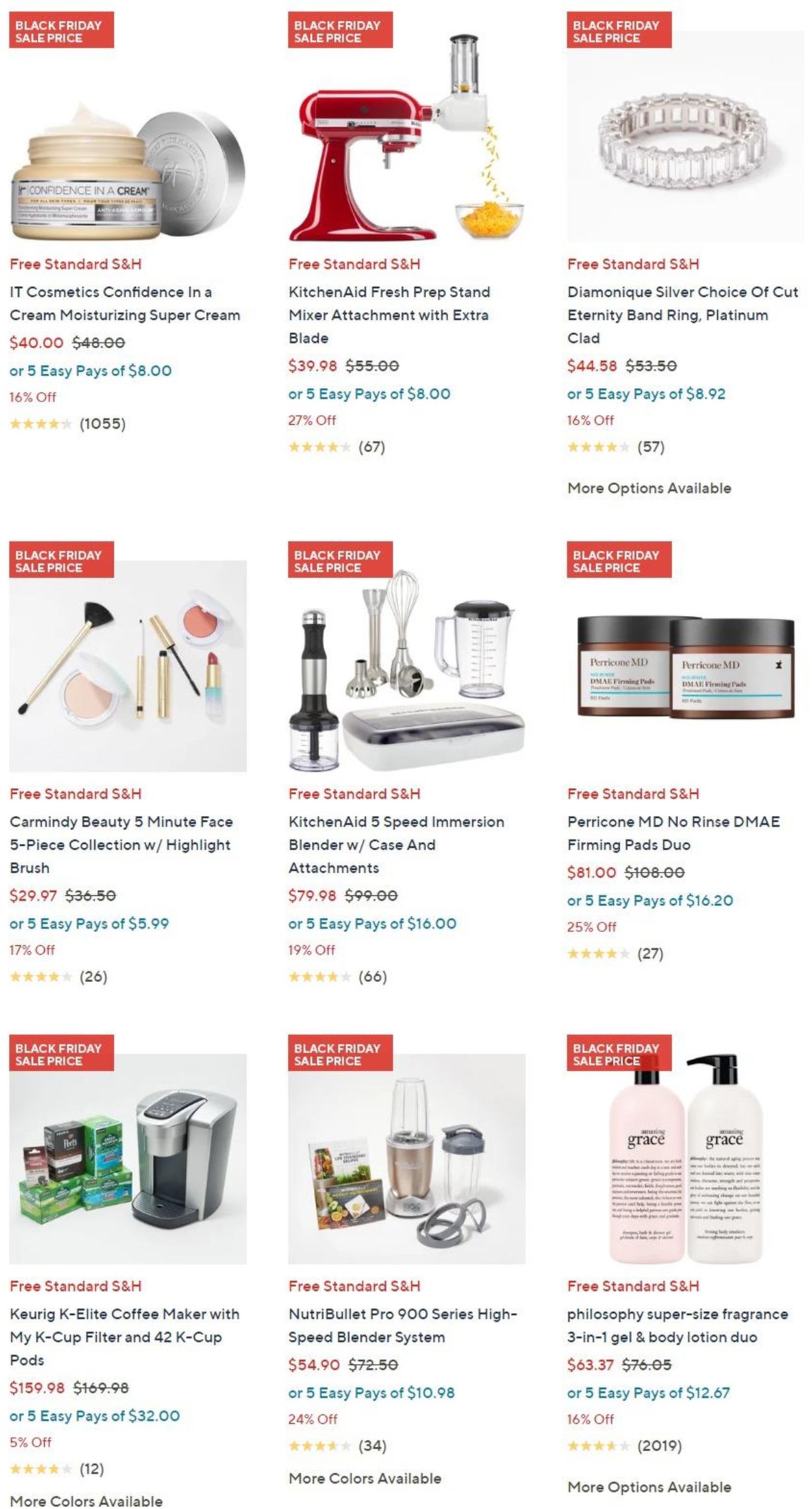### Detailed Caption for a 3x3 Sale Items Chart Image:

This image showcases a 3x3 grid of various items on sale, prominently featuring a "Black Friday Sale Price" banner in red at the top of each entry.

**Top Row (Left to Right):**
1. **IT Cosmetics Confidence in a Cream Moisturizing Super Cream**: Displaying a price tag of "5 easy payments of $8" alongside a rating represented by stars, and indicating free standard shipping and handling. The product image features a small jar of the cream.
2. **Spiralizer (Red)**: A device designed to turn vegetables into string-like noodles, perfect for making healthy meals.
3. **Platinum Clad Band**: A sleek and elegant band made from platinum, ideal for special occasions.

**Second Row (Left to Right):**
1. **Makeup Set**: This collection includes several cosmetic items such as brushes and lipsticks, providing a comprehensive makeup solution.
2. **KitchenAid 5-Speed Immersion Blender with Case and Attachments**: A versatile kitchen appliance complete with its case and various attachments, perfect for blending, mixing, and pureeing.
3. **Perricone MD No Rinse DMAE Firming Pads Duo**: The image features two bottles of firming pads designed to tone and tighten the skin.

**Bottom Row (Left to Right):**
1. **Keurig K-Elite Coffee Maker with My K-Cup Filter and 42 K-Cup Pods**: A high-performance coffee maker packaged with a reusable K-Cup filter and 42 coffee pods for a rich brewing experience.
2. **Nutribullet Pro 900 Series High-Speed Blender System**: This high-speed blender system is designed for efficient blending, suitable for making smoothies and other nutritious beverages.
3. **Philosophy Super Size Fragrance 3-in-1 Gel and Body Lotion Duo**: A luxurious duo consisting of a 3-in-1 gel for hair, face, and body, along with a hydrating body lotion.

Each of these items is neatly arranged, clearly priced, and visually appealing, making it easy for potential buyers to compare and choose the best deals during the Black Friday sale.